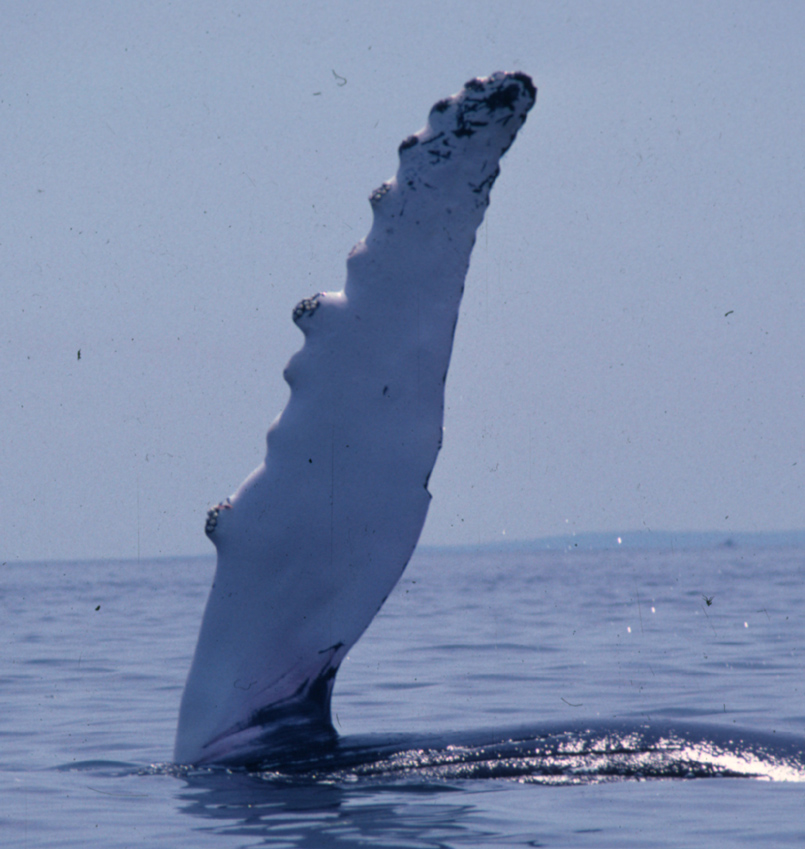This captivating outdoor image showcases the majestic scene of an ocean with a striking whale fin emerging from the water. The upper half of the photograph features a slightly grayish, yet bright sky, creating a serene backdrop void of visible sunlight. Far in the distance, a faint outline of a hilly landscape can be discerned. Dominating the lower third of the image is the ocean, its surface hinting at a subtle glare likely caused by the hidden sun.

The primary focus of the image is a colossal, jagged whale fin, which stretches almost vertically from the bottom to the top of the picture. The fin is predominantly white with a rugged texture and numerous bumps, approximately ten, lining its edge. To the right of the fin, just at the water’s surface, the black hump of the whale’s body is partially visible, hinting at its immense size. The fin's striking prominence is accentuated by some slight, possibly camera-induced, white spots scattered toward the right side of the image. Combining the soothing yet dramatic elements, the picture beautifully captures the grandeur and grace of marine life.